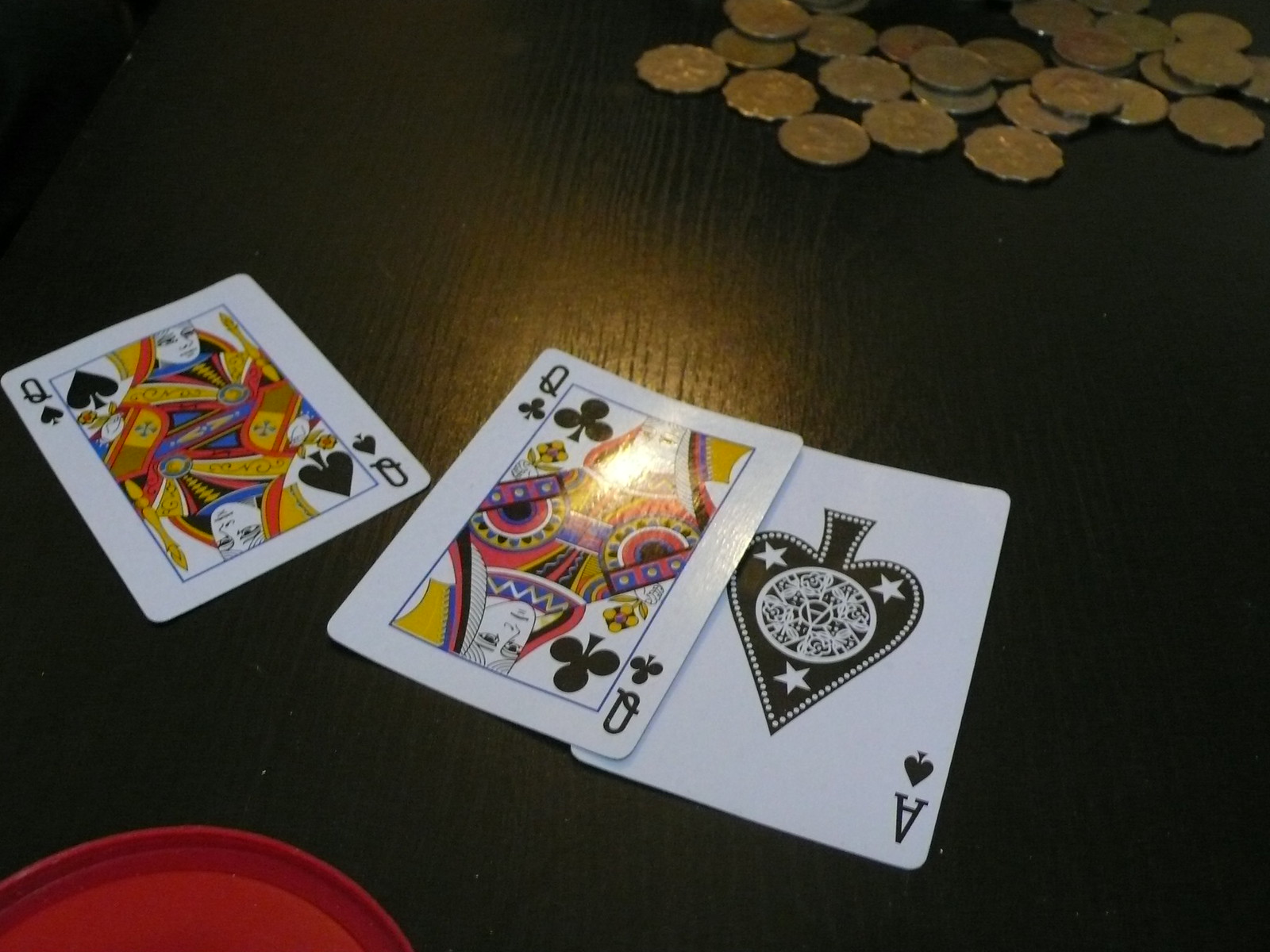A detailed close-up photo captures an intense moment in a card game in progress, played on a vertically-grained brown wooden table. The table's center is illuminated by a bright light, creating a shiny surface that adds a slight glare. In the upper right-hand corner, a pile of approximately 25 gold coins with scalloped edges suggests a currency unfamiliar to the observer. These coins are clustered together, with a few scattered individually. In the lower left-hand corner, partially visible, is the underside of a red Tupperware lid. The central focus of the image is on three playing cards against a white background. The Queen of Spades stands alone to the left, while the Queen of Clubs is slightly tilted to the right, overlapping the Ace of Spades. The bright light enhances the visibility of the Queen of Clubs, although it casts a glare on her head, obscuring her facial features.